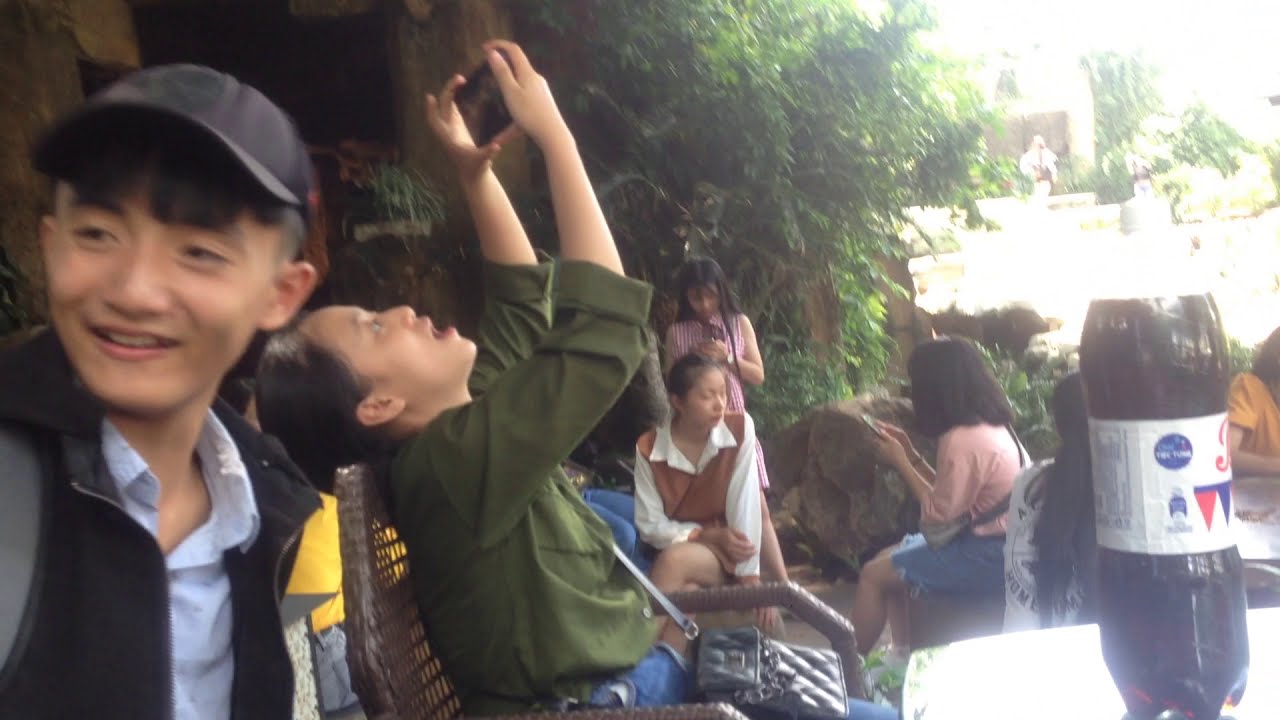In this outdoor photograph, several people are gathered, primarily on the left side of the image and extending through the center. To the far left stands a young Asian boy, smiling, wearing a black baseball cap, a light blue collared shirt, and a black vest. He is looking slightly frontward but turned to his left. Directly to his right is a girl in a long-sleeved, rolled-up olive green shirt and blue jeans, with a black crossbody bag that has cushioning on the surface. She appears to be leaning back over a park bench, looking up at her smartphone as she possibly takes a selfie. The scene is bathed in bright sunlight, evident in the top right corner of the image. In the foreground to the right, a bottle of dark-colored soda with a white label featuring red and blue triangle designs and a blue circle with unreadable white text sits on a table. In the background, several other people, including some younger children, can be seen among the trees, highlighting that this setting is likely a park and suggesting it could be somewhere in an Asian country. The colors in the image include shades of brown, black, tan, light blue, yellow, green, gray, white, and red, contributing to the lively atmosphere.